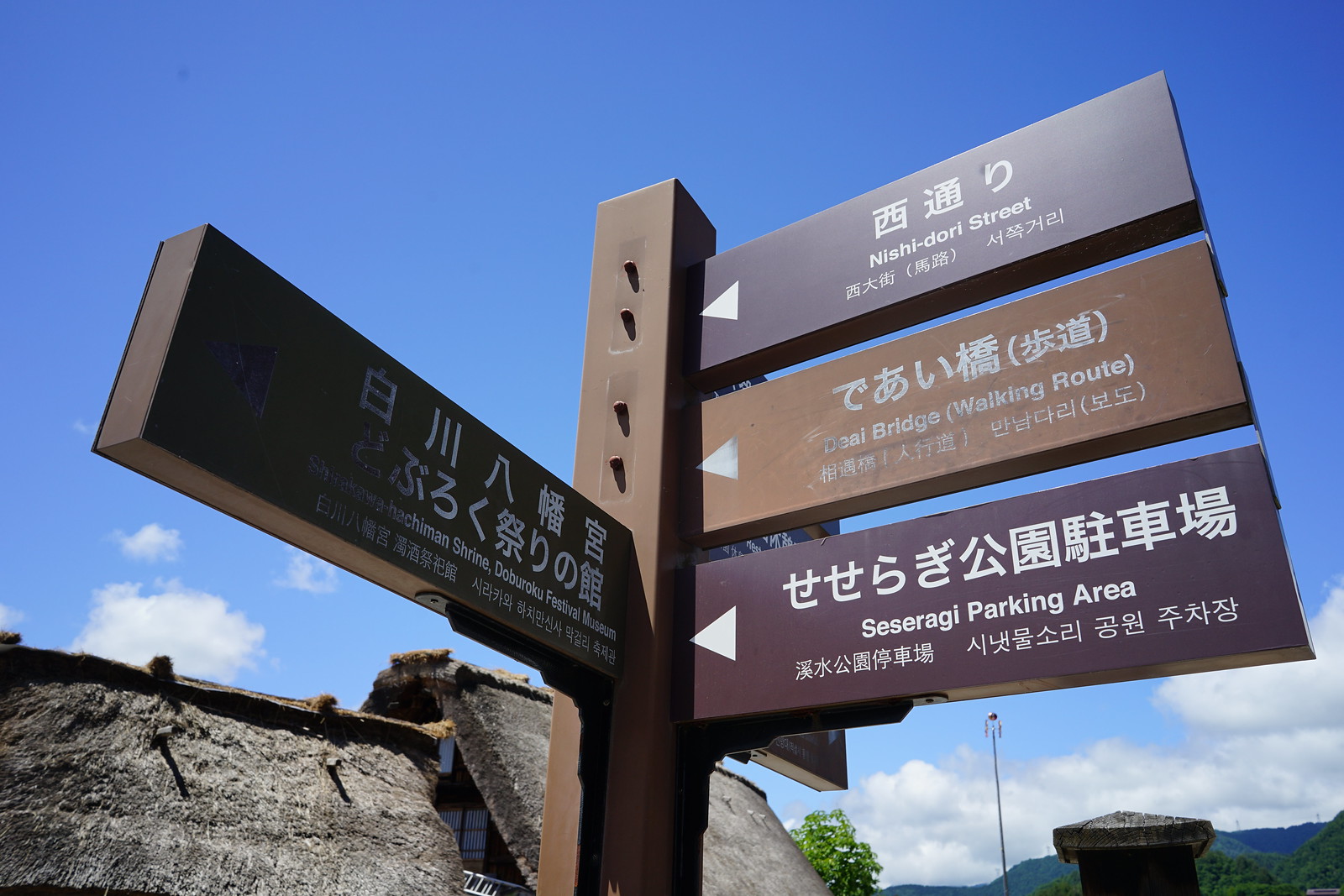This photograph, taken outdoors on a partly cloudy day with blue skies and low-lying clouds, features a wooden directional marker situated in front of what appears to be an old, historical fort, possibly located in a Far Eastern region, likely Korea or Japan. The signpost, shown in remarkable clarity, has multiple directional planks pointing to various locations. There are three signs on the right side, all with arrows pointing left, and one partially obscured sign on the left. The top sign on the right reads "Nishidori Street" with Japanese characters above the English translation. Below it, another plank indicates "Daiyo Bridge walking route," and the third one directs to the "Seseragi parking area." The left plank, shaded due to the sunlight coming in from the left, mentions "Hachiman Shrine" and "Doboroku Festival Museum." The background reveals the fort's parapet and walls, topped with roofs of two larger buildings to the left and a smaller structure to the right. The overall scene is dominated by a vivid blue sky and distant greenery, suggesting a blend of historical intrigue and natural beauty.